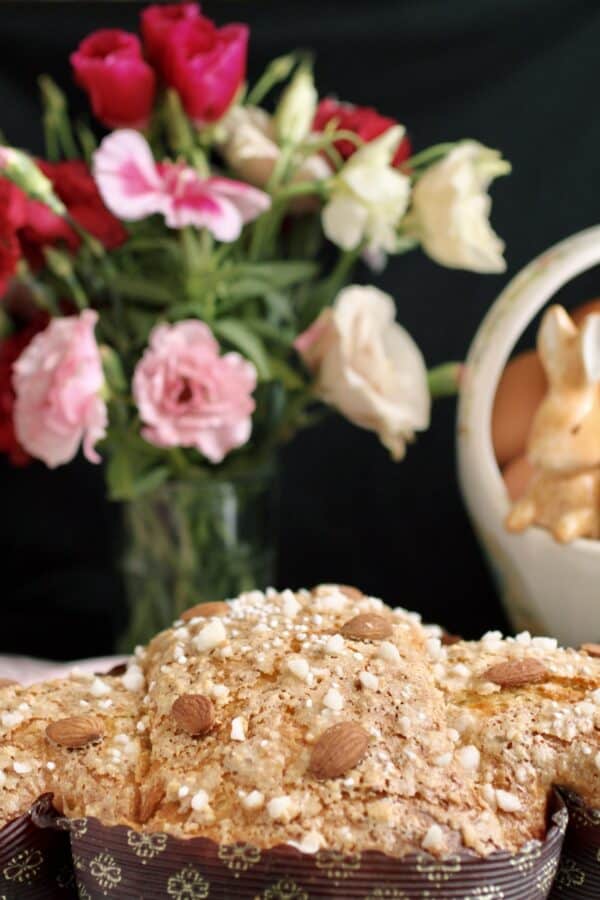This vibrant color photograph captures an inviting scene with multiple elements. In the foreground, a collection of baked muffins, nestled in distinctive brown paper wrappings adorned with gold cross designs, draws immediate attention. Each muffin features a crumbly surface generously sprinkled with areas of pearl sugar and slivered almonds. The background showcases a bouquet of delicate roses in various shades of pink and white, elegantly arranged in a clear glass vase. Adjacent to the vase, a white ceramic Easter basket sits, cradling a tan-colored ceramic rabbit. The setting is contrasted against a black backdrop, allowing each element to stand out vividly.